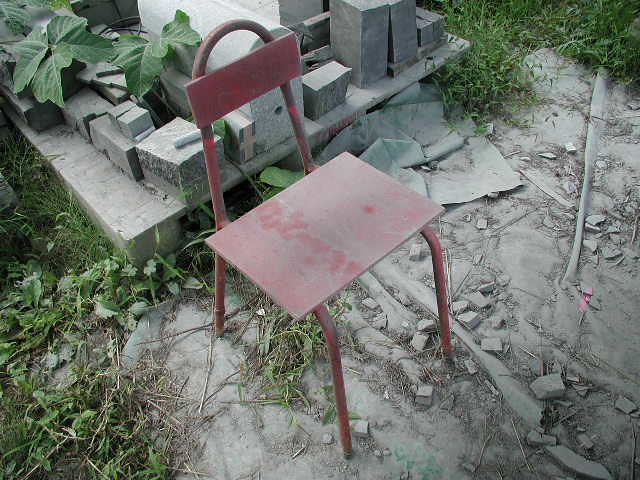This horizontal rectangular image captures an outdoor scene where an old, rusty red metal chair, likely homemade, stands as the central object. The chair, with its flat metal seat and back supported by metal legs, appears uncomfortable and significantly weathered. It rests on a crumbling concrete slab surrounded by a blend of loose stones, old, dead weeds, and patches of grass. A concrete platform behind the chair holds scattered, abandoned bricks and cinder blocks, suggesting an unfinished or neglected construction area within a garden or patio space. The entire setting is well-lit by natural daylight, highlighting the contrast between the red chair, the gray concrete, and the surrounding greenery.